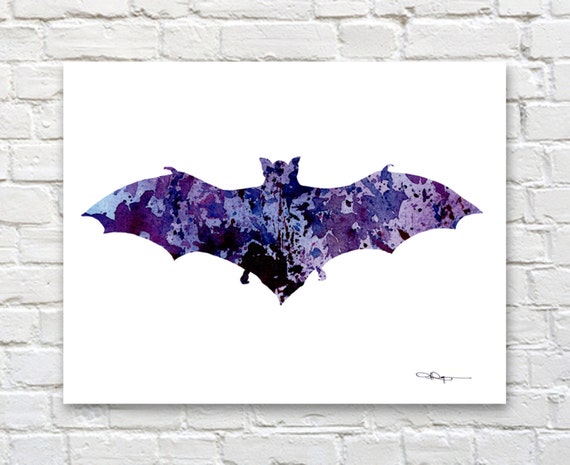This image features a detailed painting of a bat with its wings spread, displayed on a white canvas. The bat's back view is showcased, with the body predominantly painted in various shades of purple, including lavender, violet, and other hues such as black, blue, and grey, dispersed randomly across the wings and body. Symmetrically designed, the silhouette of the bat includes visible ears and small legs. A loopy, cursive black signature is located at the bottom right corner of the canvas. The entire artwork appears to be superimposed onto a background of a white, rectangular brick wall, complete with a drop shadow that suggests it has been digitally manipulated rather than physically attached.